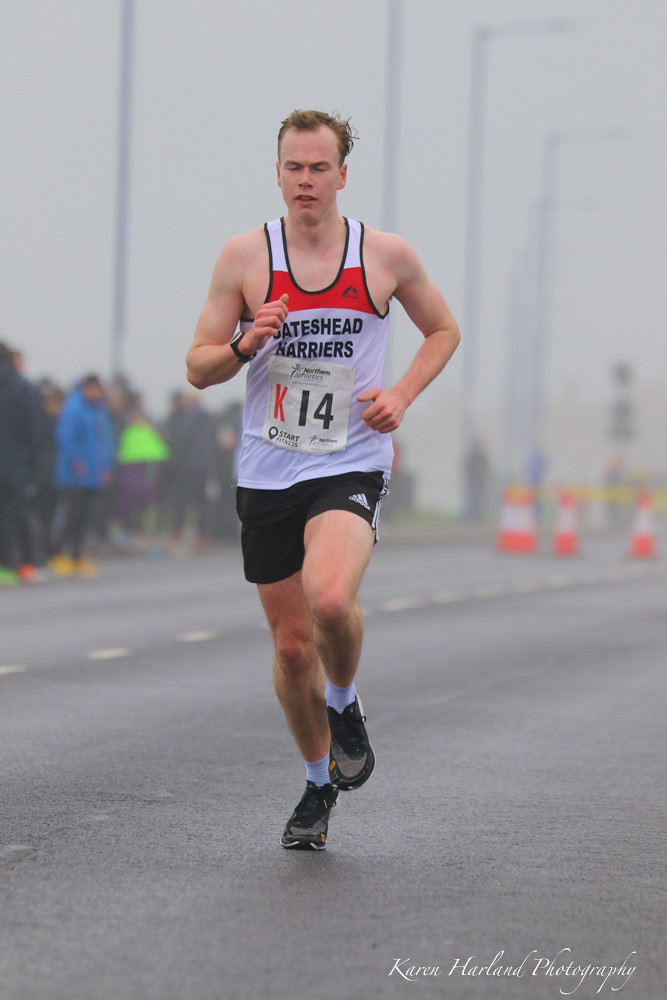In this captivating photograph, a Caucasian man is captured in mid-stride as he runs a marathon in the rain, his fatigue evident in his closed eyes and disheveled hair. Dressed in a white tank top that clings to his sweat and rain-soaked skin, the tank top features an orange band around the top and a distinctive red stripe down the center. His race bib, which reads "K14" in black text, is securely attached to his shirt, bearing the logo of the "Gateshead Harriers," likely his sponsoring club. The runner's lean physique displays defined muscles in his arms, complementing his black Adidas shorts, grey sneakers, and white socks. He also sports a black watch on one wrist. The background is a blur of grey, foggy ambiance, accentuated by spectators lining the street in winter attire, umbrellas, and rainproof clothing, indicative of the cold and rainy weather. They stand on the left side of the image, beside a bridge, as the runner perseveres through the dreary conditions. The photograph, tagged as "Karen Harlan Photography" at the bottom, skillfully captures the lone runner in focus, set against a hazy, cone-marked street, illustrating both the physical challenge and the atmospheric elements of the marathon.